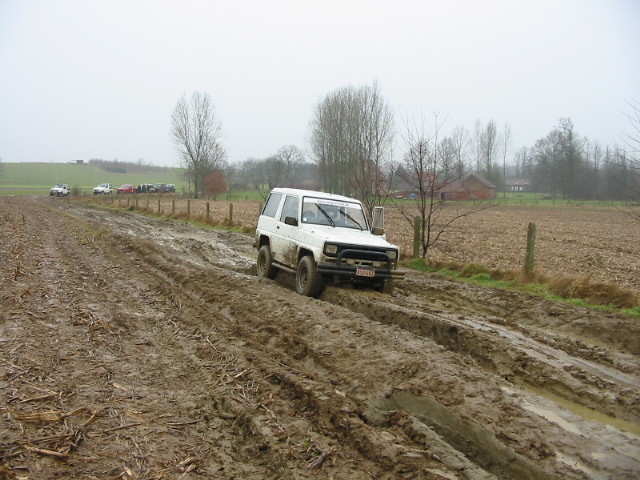This image depicts a white SUV, possibly a Ford Bronco or jeep, struggling in a muddy, rutted track amidst what appears to be a desolate, possibly winter or fall, farmland area. The SUV has its doors open, suggesting attempts to escape from the thick mud, which seems about a foot deep in some places. The setting includes a few scattered houses and farm trucks, with a background featuring trees, a green mountainside to the left, and a few additional vehicles about 900 feet behind, indicating there might be some kind of farming event or competition. The sky is gray, adding to the overall bleak, muddy ambiance, reminiscent of a family's challenging yet typical day on a farm.